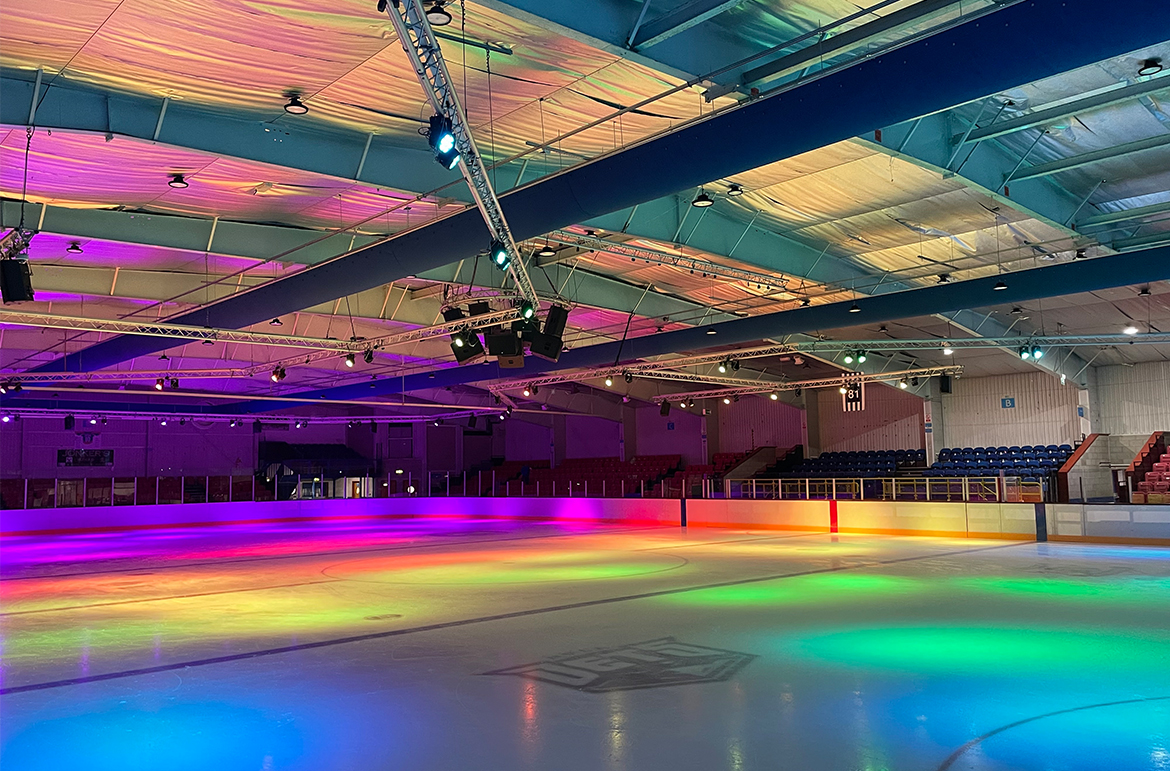This photograph captures an empty indoor ice rink, which appears to be set up for a light show. The rink features multi-colored neon lights that project vibrant hues such as magenta, purple, red, orange, yellow, lime green, turquoise blue, and soft blue onto the ice surface. The absence of fans or players indicates that this visually striking display is intended purely for decorative purposes. The ice itself showcases a logo, possibly reading "Jets," and has a diamond-shaped outline. The arena is large with a tall ceiling supported by beams, and the divider walls around the rink are half-height with plexiglass on top. Seating is visible on the right side, including blue and red chairs in the stands, possibly indicating different seating sections. Additional elements like scaffolding, speakers, and black lamps for the lighting setup can also be observed, enhancing the overall ambiance of the scene.